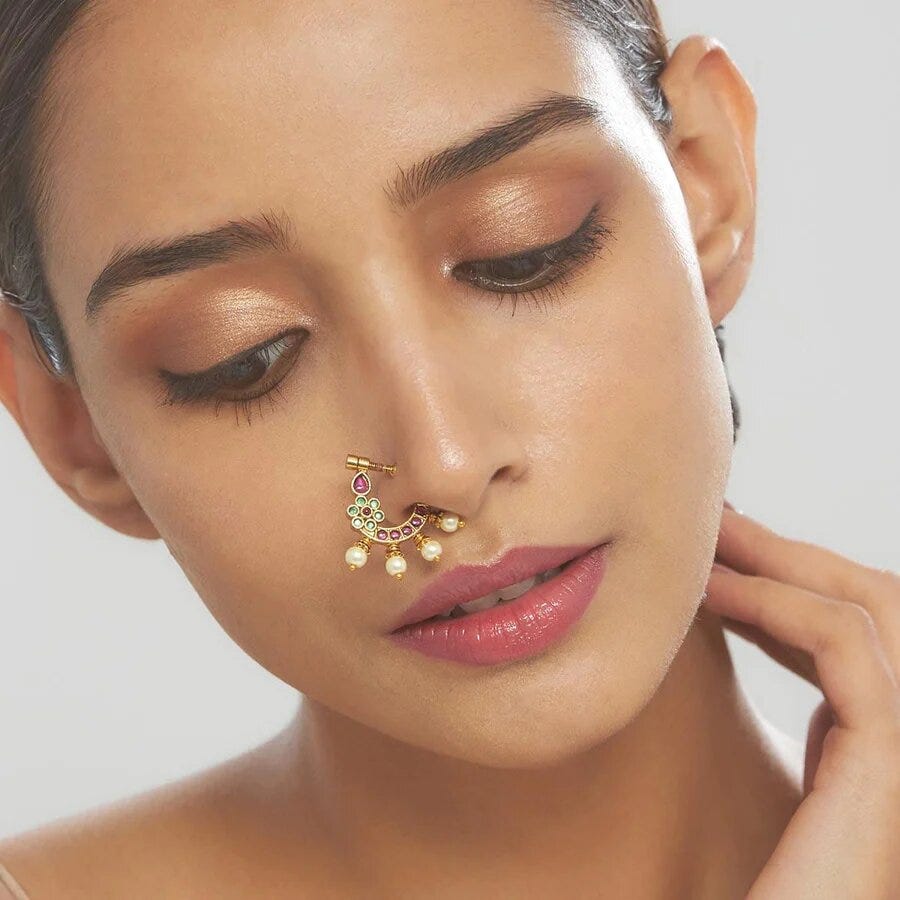This high-resolution, indoor, square-format photograph captures a beautiful young woman of South Asian descent with an Indian appearance, likely in her late teens to early twenties, in a contemplative pose. She has a fair complexion, clear skin, and dark hair pulled back off her face. Her delicate features include dark eyebrows, long eyelashes framing her brown eyes, and a Caucasian-like nose. She is adorned with subtle makeup, sporting shimmery shell-pink eyeshadow, lightly tinted pink lips, and a striking nose ring in her left nostril. This ornate nose ring features a pink teardrop gem and a green gemstone flower, with four pearls extending from prongs at the base, forming a hoop that arches up into her nostril. Her lips are slightly parted, revealing her teeth, and she glances downwards to her right with her left hand gently pressing against her neck, emphasizing her serene and reflective expression. The close-up shot primarily focuses on her face, neck, and part of her shoulder, with the top of her head cropped out of the frame.